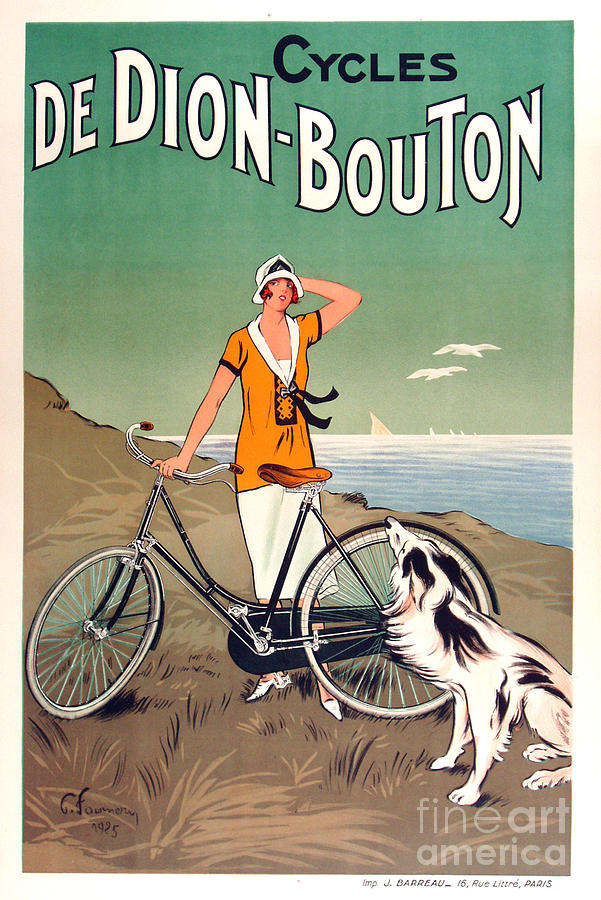The image depicts a vintage magazine cover from the 1920s, rectangular in shape and measuring approximately 5 to 6 inches high by 3 inches wide. It features a thin border with a white top and bottom and pale tan or peach tones on the left and right sides. Dominating the cover, the top half showcases a sky that transitions from green to a yellowish-green near the horizon. In bold black print at the upper right, the title "Cycles" is displayed, followed by "De Dion Bouton" in bold white print with a black outline.

Below the horizon line on the right, a serene blue bay with white sailboats and birds is visible, adding a tranquil touch to the illustration. The left side highlights a brown, grassy hill upon which a young Caucasian woman stands beside her bicycle. She sports short brown hair and a white flapper-style hat, indicative of the 1920s. Her attire consists of a long, orange tunic-style shirt with a V-neck, a white skirt, and matching white shoes. At her feet, a small white dog with patches of black fur gazes up at her.

This detailed artwork, possibly signed by an artist with a name resembling "G. Foamy," dates back to 1925. It captures a nostalgic seaside scene complete with sailboats, seagulls, and a rocky, grassy cliff, evocative of early 20th-century advertising or movie posters.